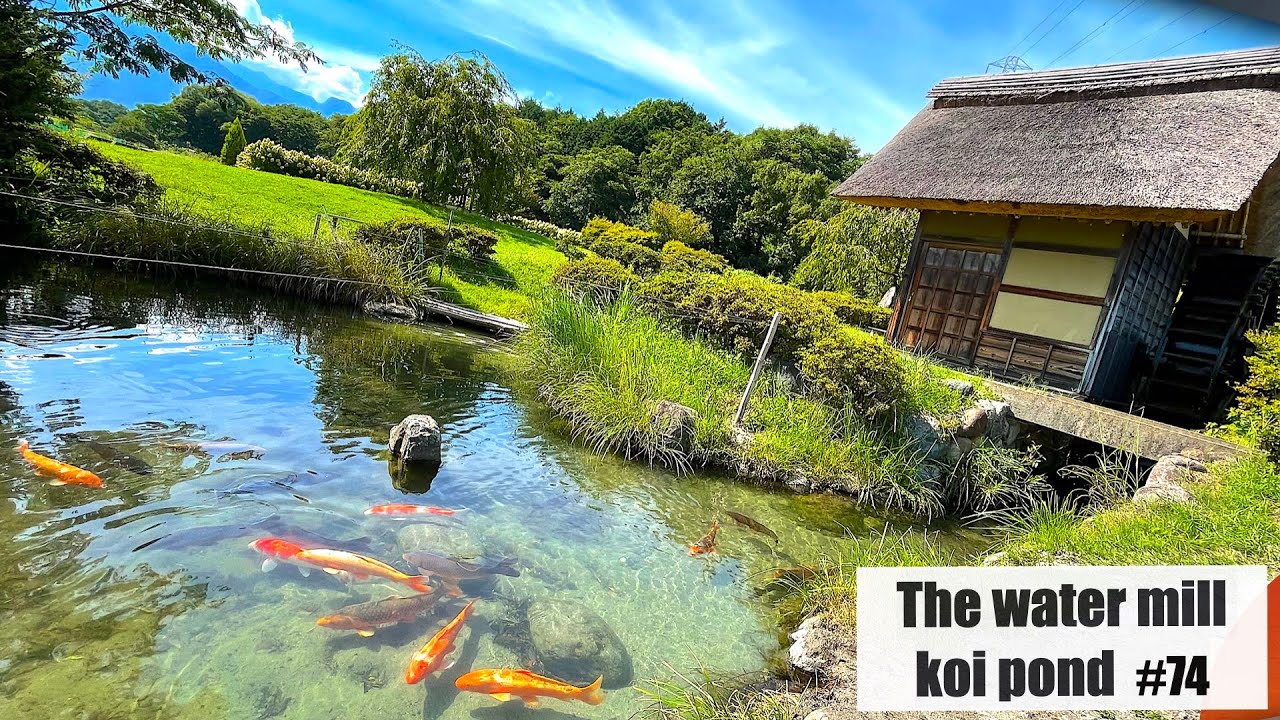This daytime outdoor photograph, measuring six inches wide by about three inches high, showcases the Watermill Koi Pond, labeled "number 74" in bold black print on a small white rectangle located in the lower right-hand corner. Adjacent to this label is a distinctive red semicircle. Prominently featured in the center and left of the image is a clear water pond teeming with golden and white koi fish swimming over a bed of rocks. The pond is bordered by an array of green shrubs, long grass, and gray rocks both in and out of the water, contributing to the naturalistic setting. 

Emerging from the right side of the photograph and extending upward to the left is a small, rustic house, reminiscent of a Japanese mill. This structure, seemingly fragile with its weathered wooden frame and natural grass-thatched sloping roof, rests atop a stone platform that also serves as a bridge over a section of the pond. The background features a well-maintained field of green grass, interspersed with trees, under a bright blue sky dotted with white clouds. An almost hidden wire runs along the edge of the pond, presumably installed to prevent people from falling in. Overall, the scene exudes a serene, natural charm, capturing the vibrant yet tranquil environment of the Watermill Koi Pond.